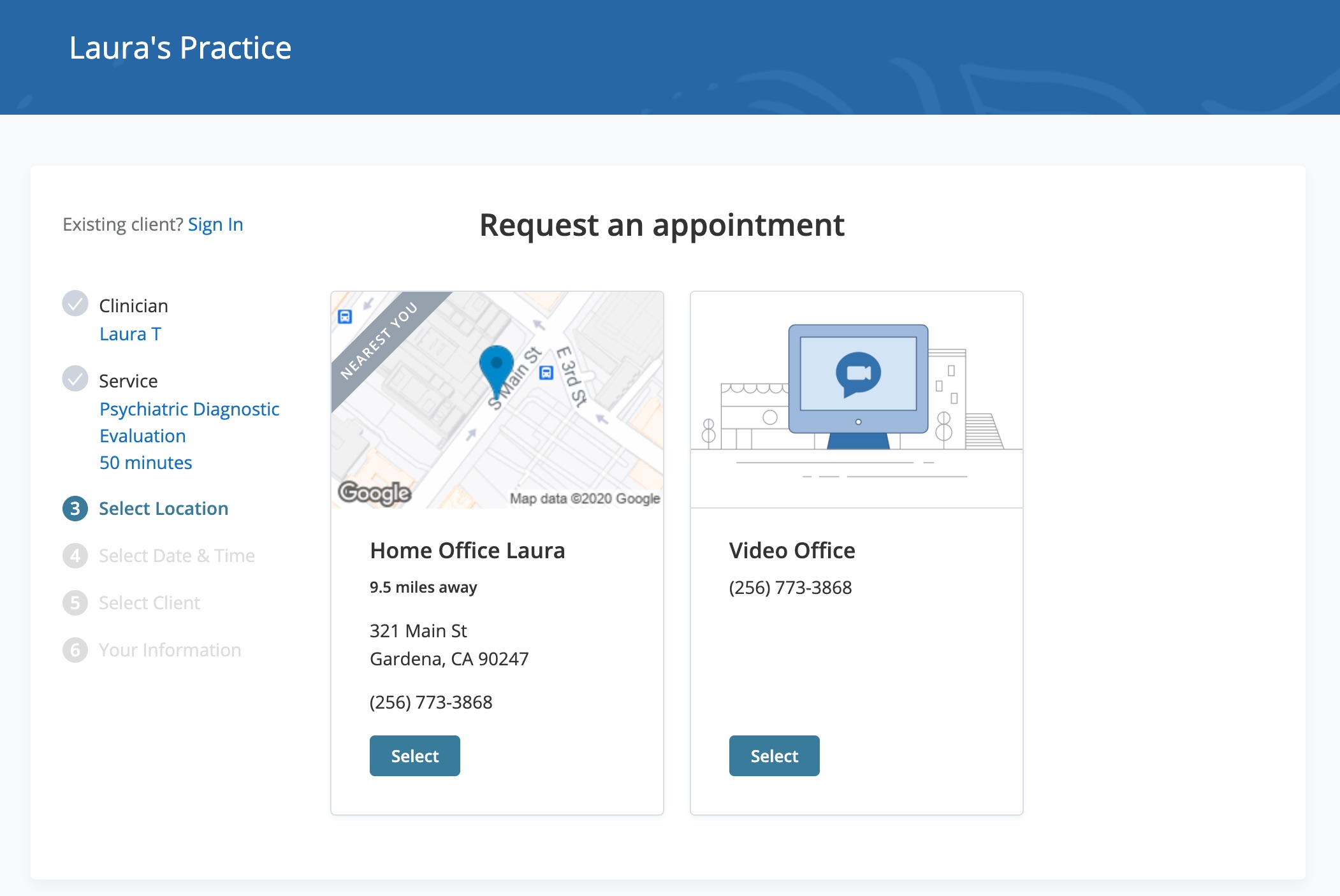**Detailed Caption:**

The screenshot displays the interface of a scheduling platform for "Laura's Practice." The light blue top bar prominently features the text "Laura's Practice" in white font. Just beneath it, there's a black header stating "Request an Important Appointment" against a white background that extends throughout the screen.

On the left side, a light gray text reads "Existing Client?" with a blue "Sign In" option to its right. Below this, a section titled "Clinician" is listed, showing "Laura T" in blue with a checkmark inside a gray box on the left. 

Following that, there's another checkmark within a gray circle next to the word "Service." Under the service section, "Psychiatric Diagnostic Evaluation - 50 minutes" is written in blue. The third highlighted element is "Select Location," enumerated as step three, set against a blue background.

Further below, gray and faint step indicators 4, 5, and 6 can be seen, but their labels are unreadable due to their light coloring. The "Select Location" section displays a black-and-white map with a pinpoint marked in blue. The map includes the attribution "Google" and a copyright notice, "Map data ©2020 Google."

Beneath the map, two options for appointment locations are provided:
1. **Home Office:** Listed as "Laura, 9.5 miles away," located at "321 Main Street, Gardenia, California, 90247," complete with a phone number and a blue "Select" button.
2. **Video Office:** Depicted with an animated computer screen and a video camera icon, set against an animated cityscape. Below this, it says "Video Office" in black text, displays the same phone number, and features another blue "Select" button.